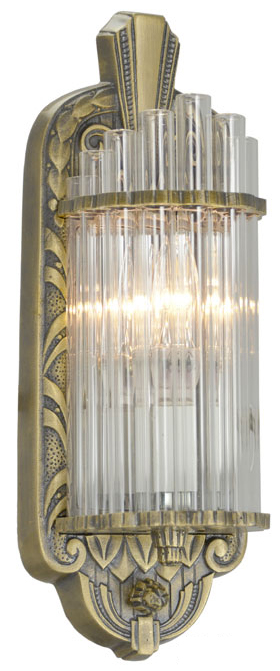This image features a highly ornate sconce set against a completely white background. The sconce itself is composed of a brassy gold base with darker, brushed gold tones and intricate leaf designs and swirling patterns at the bottom. The upper section of the sconce includes a raised point that adds to its elaborate appearance. The light is enclosed within a series of glass tubes, which vary slightly in height—taller in the middle and shorter on the sides. These tubes are held in place at the top by a gold ring, giving a structured yet elegant appearance. The light within emits a white-yellow hue, visible as a thin horizontal line through the transparent glass tubes. The sconce is oriented slightly towards the right, showcasing only one side in detail.